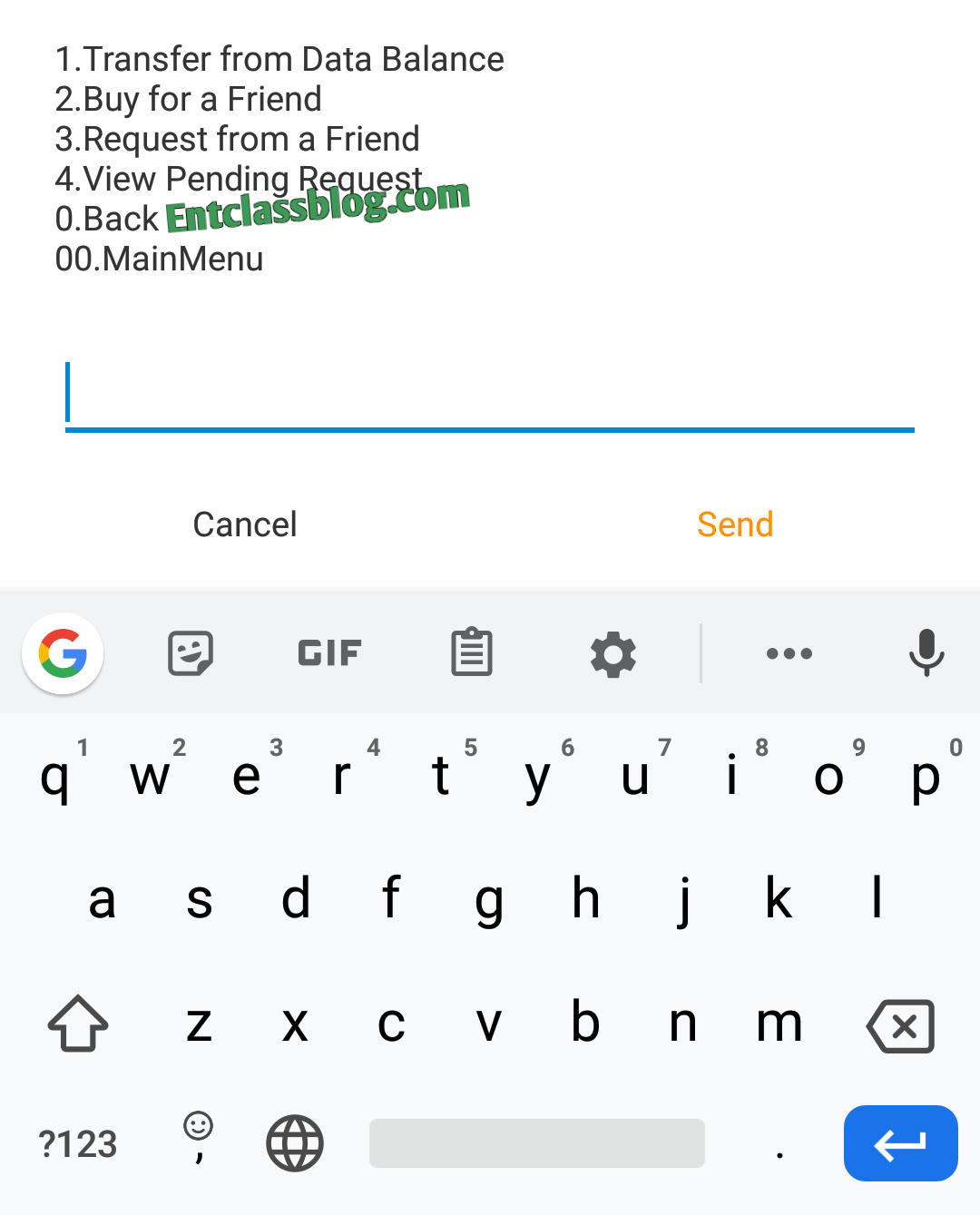An up-close screenshot of a smartphone interface reveals a detailed menu without the top status bar displaying battery, time, or signal. The screen showcases several options numbered sequentially: 
1. **Transfer from Data Balance**
2. **Buy for a Friend**
3. **Request from a Friend**
4. **View Pending Requests**
   
A heading at the top reads "0.0" and a "Back" button. Diagonally across the screen, the text "NTClassBlog.com" is written in green. Below this, a primary label "MAINMENU" is displayed in capital letters, underneath which a blue line separates it from other content. Following this, there are "Cancel" (in black) and "Send" (in gold) action buttons, both in the same font size.

Below the buttons, a bar contains various icons: a Google icon, a smiley face on a sheet of paper, a GIF icon, a clipboard, settings icon, three vertical dots for more options, and a microphone. The QWERTY keyboard appears at the bottom, featuring a row of numbers across the top. Despite the informative layout, the purpose of this interface remains unclear.